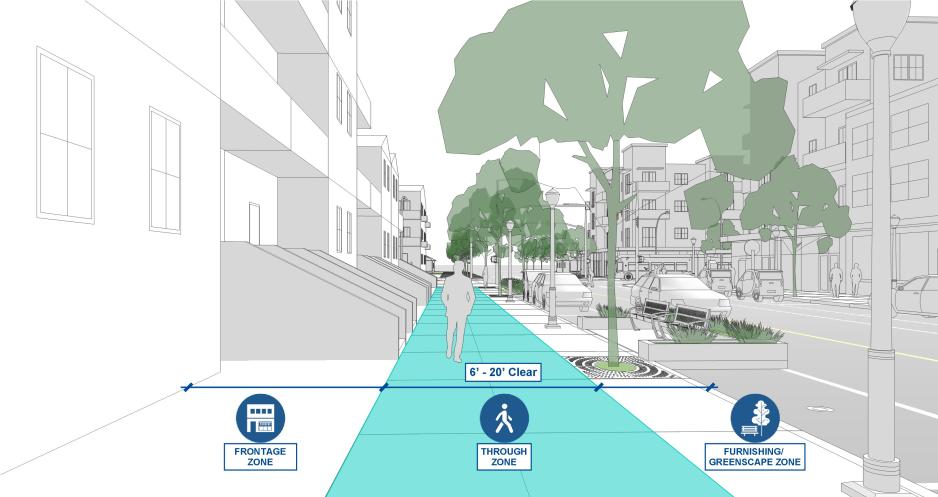This computer-generated image depicts a city street from a horizontal, rectangular perspective without a border. The scene shows a mix of detailed elements and colors: a mostly white background where the sky and left-building regions are, contrasting with various shades defining other aspects of the street. On the left, there's a white building with windows and a white sidewalk beside it. Extending from the center bottom towards the middle of the image, there's a light blue sidewalk with a gray outline of a person walking on it. Adjacent to this sidewalk, between it and the street, is a white section dotted with green trees. This white area also continues into the distance with more trees appearing as you look further up.

In the middle-left to the center top, there's a green section of the sidewalk leading into the image. The right side features a gray street with gray cars. Across the street are more gray-shaded buildings with cars parked along the side. A gray light pole is positioned at the bottom right of the image, highlighting additional infrastructure. 

A horizontal blue measurement line spans across the image, intersecting the sidewalk and white areas, labeled "six feet - 20 feet clear". At the bottom, three small icons are visible: the left icon displays a building labeled "Frontage Zone," the middle icon shows a person labeled "Through Zone," and the right icon features a bench and tree, labeled "Furnishing / Greenscape Zone." This elaborate and structured layout suggests that the image is a detailed city planning diagram.